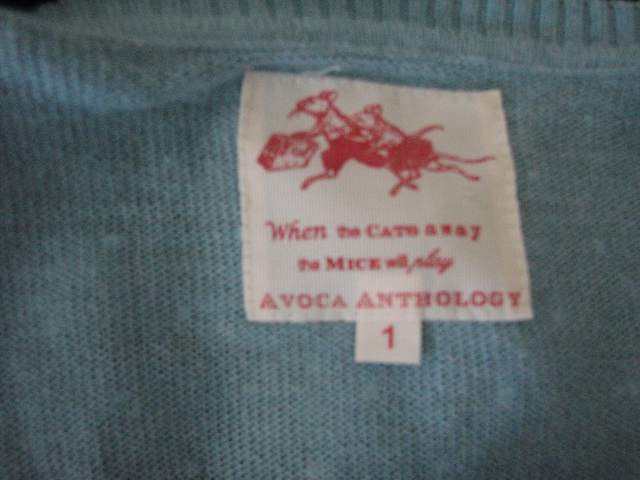This close-up image captures the tag inside the neckline of a finely knit blue garment with a ribbed neck. The tag is white with red printing, featuring an animal emblem that is somewhat indistinct and out of focus. The text on the tag reads, "When the cat's away, the mice will play," with some words displayed in cursive and inconsistent fonts. Below this text, the tag lists "AVOCA" and "Anthology." Additionally, there is a smaller tag attached, displaying the number "1."